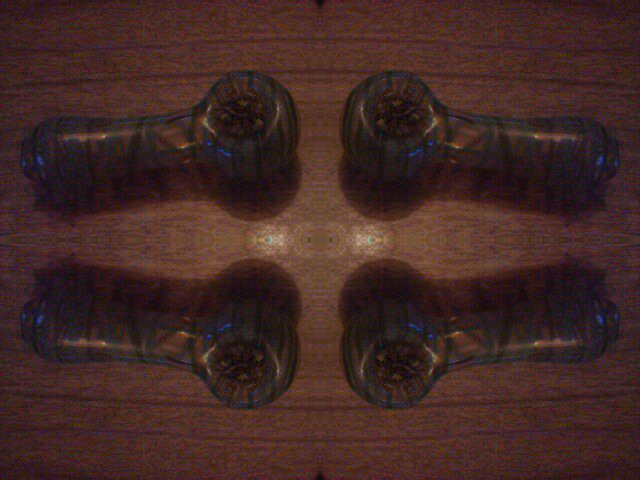This image is a close-up of four identical, ancient-looking tools arranged symmetrically on a dark wooden table. The table has a medium brown tone with darker etched lines and visible grain, illuminated slightly by reflective light. The tools are constructed of metal and exhibit a dark brown to black coloration with some tan, reminiscent of a camouflaged pattern. Each tool features a short handle attached to a round, bowl-like top with a central dip, resembling the bowl of a pipe. The bowls appear used, containing some packed material. The objects are positioned with two above and two below, creating a rectangular arrangement with gaps between pairs, placed bowl to bowl and handles facing outward.